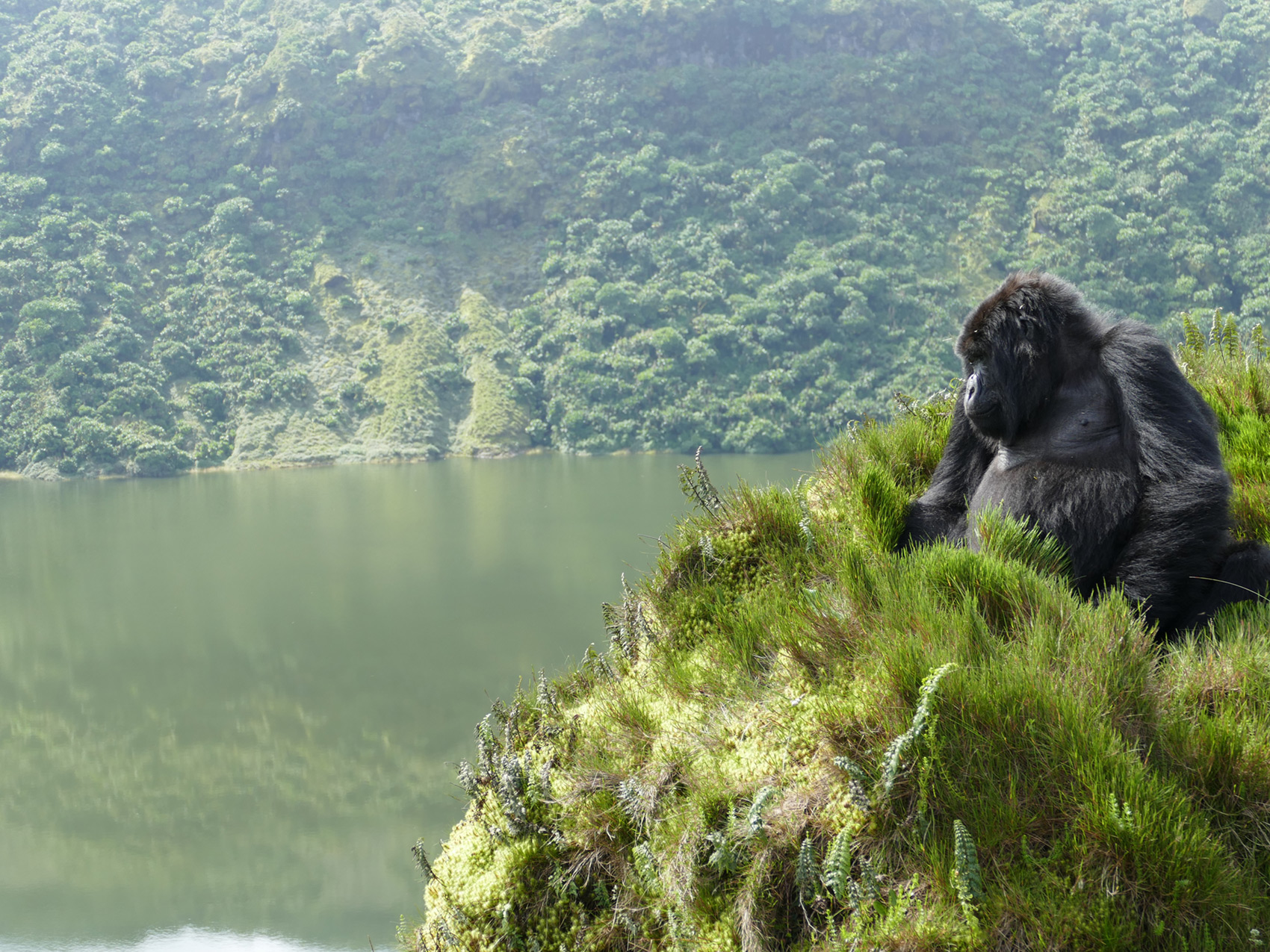In this vivid photograph of a lush forest landscape, a single female black-furred gorilla is featured prominently in the foreground, sitting majestically on a grassy green ledge. Her contemplative gaze is fixed on an olive-green lake that mirrors the surrounding scenery, possibly reflecting a range of soft hills or distant mountains. The background reveals a dense, verdant jungle composed of varying shades of green, with trees, bushes, and foliage creating a rich tapestry of life. Specks of white and tan break up the green, adding dimensionality to the landscape. The tranquil setting evokes a sense of the gorilla's natural habitat, offering a serene glimpse into wildlife in its purest form.